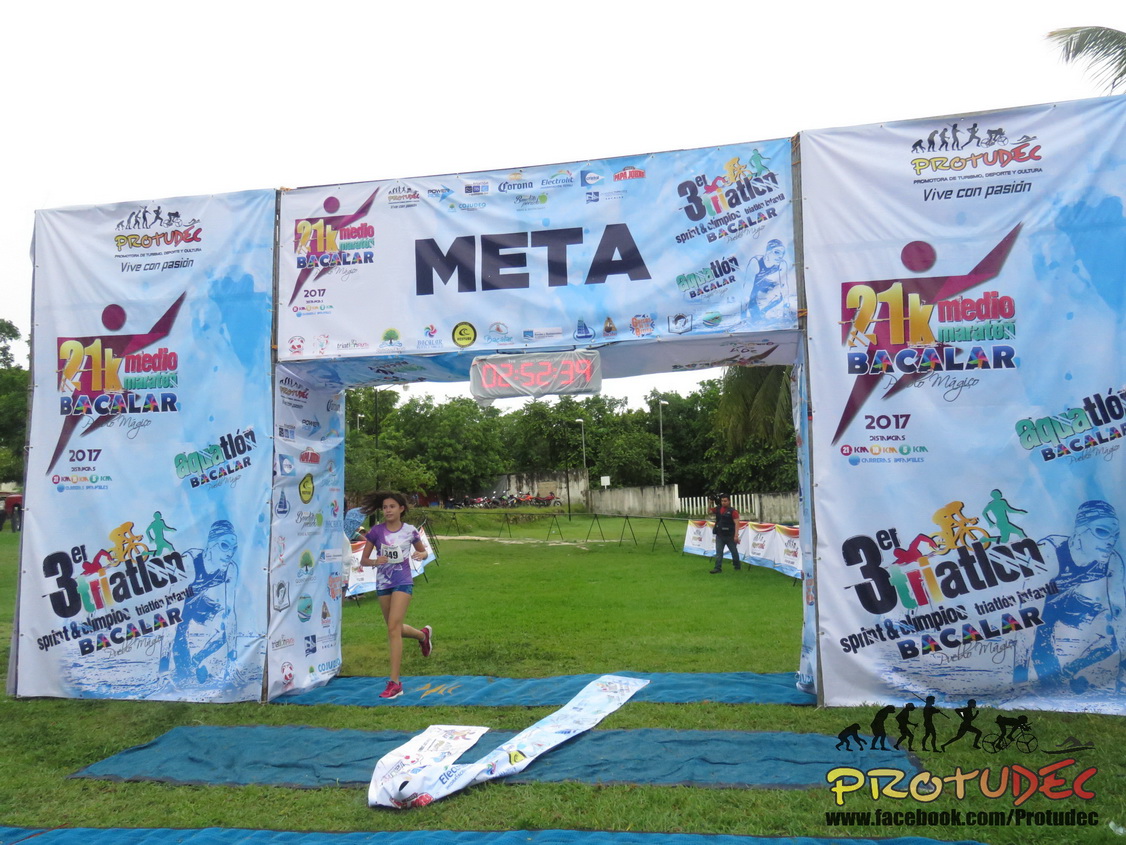A female runner, wearing blue shorts, red running shoes, and a white top, is captured mid-stride as she runs beneath a prominent archway. The archway features the word "META" at the top center, with a runner symbol representing the event. The event title is located on the right side of the archway, though the small lettering makes it difficult to read. The left and right sides of the platform display a repeated design of the central elements. Blue tarps are laid out in a line pattern on the ground, guiding the runner’s path. The image captures the dynamic energy and organization of the event, despite some textual elements being hard to decipher.